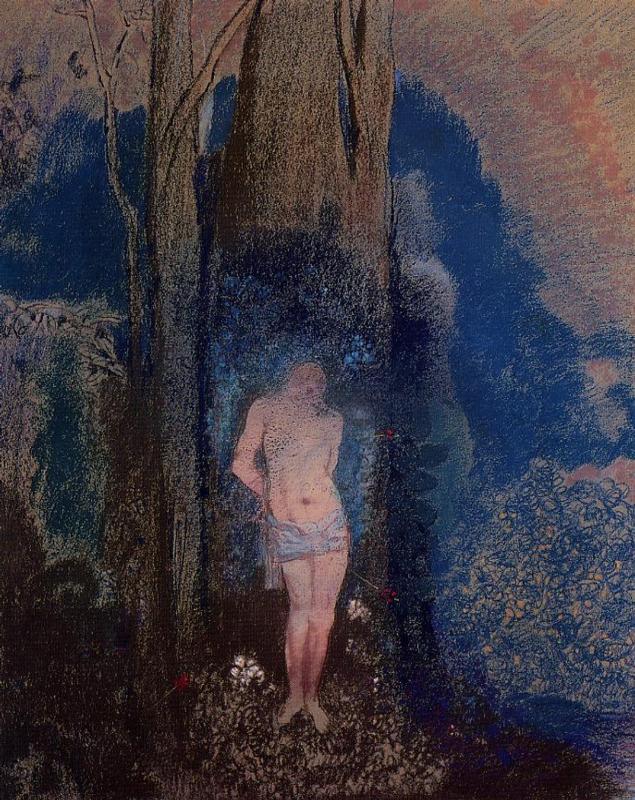This painting, in portrait orientation, features a central figure standing in front of a large, brown tree trunk. The figure, whose body is white and mostly naked except for blue-colored shorts or a loincloth, stands with joined legs and hands bound behind their back. The face of the figure is small, not very clear, and appears somewhat abnormal or smudged. The background consists of a blend of blue and light brown colors, with the blue hue seemingly representing the sky, possibly at sunrise, and casting a blue shade onto the tree. To the left of the main tree are two smaller trees growing close together. The ground around the figure is primarily brown, dotted with white and green specks, which might suggest flowers. The overall composition has an abstract quality, with smudged and dark elements, including dark blue skies and darkish clouds.